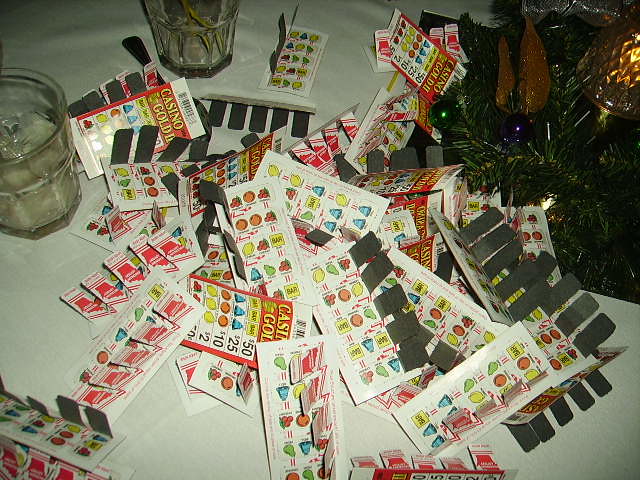The image depicts a cluttered tabletop covered with a white tablecloth, dominated by an assortment of pull-tab lottery tickets scattered haphazardly, hinting that none are likely winners. The tickets, which feature fruits like oranges, lemons, and pears, include one labeled "Casino Gold" and others with denominations such as $50, $25, $10, and $2. Toward the top left corner, two short, octagonal glasses contain a white liquid, possibly with ice. The upper right corner features a centerpiece adorned with green garland, reminiscent of Christmas decorations, suggesting the photo may have been taken during the holiday season. The image is a horizontally oriented photograph taken from above.